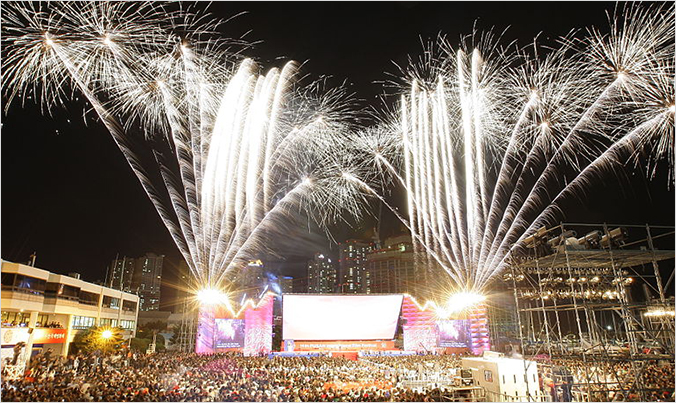The horizontal rectangular image captures a bustling nighttime scene in a stadium filled with hundreds, if not thousands, of spectators, though the playing field remains out of view. The scene is illuminated not only by the stadium lights but also by a stunning display of fireworks. These are being launched from two purple-lit areas flanking a central screen on a large billboard. The fireworks, predominantly white, include both straight vertical trails and pinwheel-like explosions. The backdrop features a dark sky dotted with tall, lit-up skyscrapers, indicating a busy urban setting. To the lower left, a beige three-story building is visible, while the lower right corner reveals scaffolding with mounted lights. The overall atmosphere suggests a concert or special event, with the dynamic and glittering display of fireworks adding a sense of festivity and excitement.